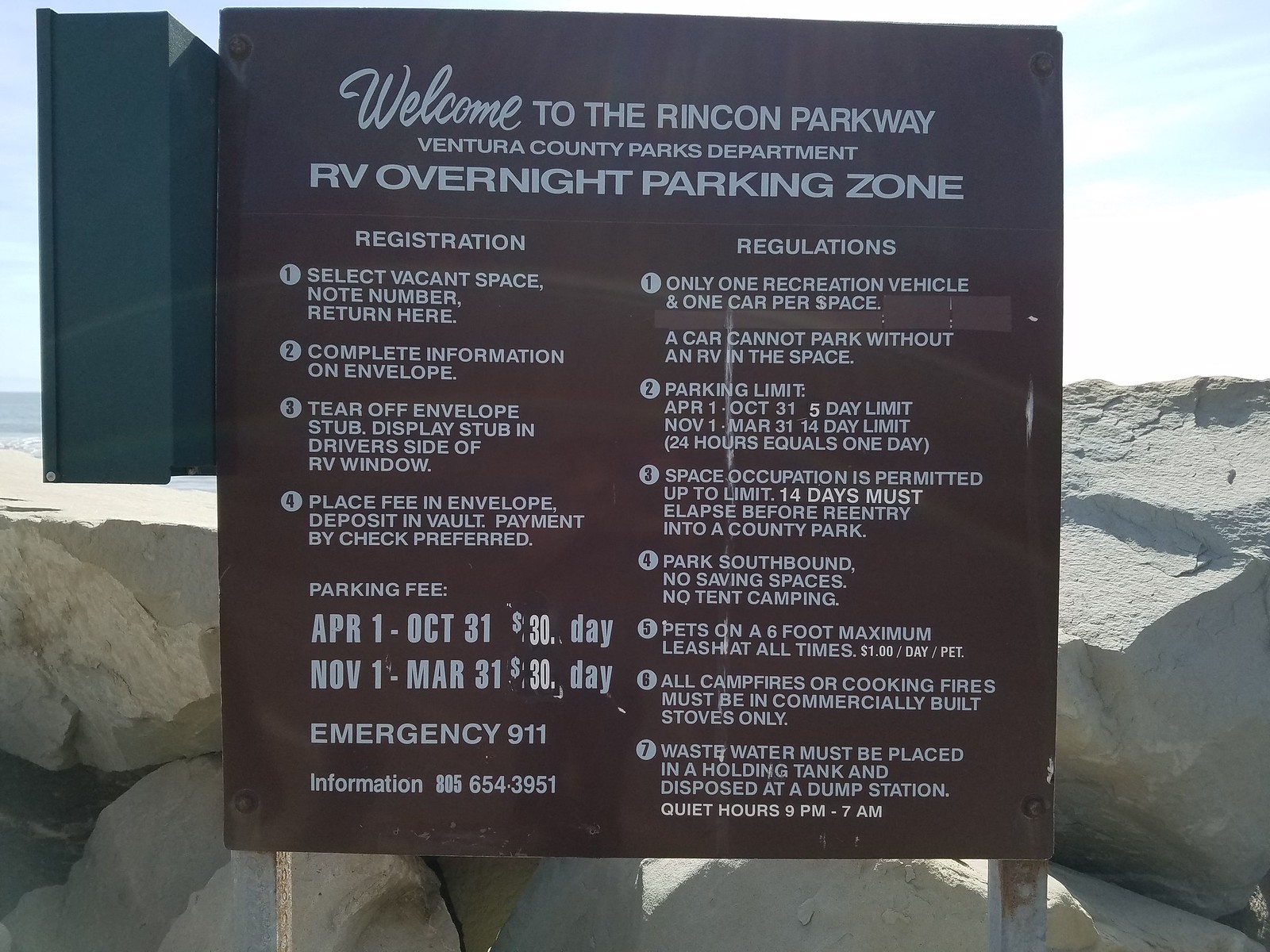This color photograph, captured in landscape orientation during the daytime, prominently features a centrally positioned, dark brown informational sign supported by gray metal posts. The close-up image, taken outdoors in a camping area, details the regulations and registration procedures for the Rincon Parkway Ventura County Parks Department RV Overnight Parking Zone. At the top of the sign, the text reads, “Welcome to the Rincon Parkway, Ventura County Parks Department RV Overnight Parking Zone.”

The left column of the sign outlines the registration steps: 
1. Select a vacant space, note the number, and return to this location.
2. Complete the information on the provided envelope.
3. Tear off the envelope stub and display it in the driver's side window of the RV.
4. Deposit the fee in the envelope into the vault, preferably paying by check. The parking fee remains $30 per day, irrespective of the months from April 1st to October 31st or November 1st to March 31st.

Emergency contact information is provided as well: dial 911, or call 805-654-3951 for further assistance.

The right column lists the regulations:
1. Only one recreational vehicle and one car per space; cars cannot park without an RV.
2. Parking limits are five days from April 1st to October 31st, and 14 days from November 1st to March 31st, with 24 hours equating to one day.
3. Space occupation is allowed up to the limit, with 14 days required before re-entry into any county park.
4. Vehicles must park southbound, and saving spaces or tent camping are not permitted.
5. Pets must be on a six-foot maximum leash at all times, with a $1 per day pet fee.
6. All campfires and cooking fires must be contained in commercially built stoves only.
7. Wastewater must be retained in a holding tank and disposed of at a dump site; quiet hours are from 9 p.m. to 7 a.m.

A blue lockbox for fee payment is affixed to the upper left corner of the sign. Below the sign, large gray boulders form a natural background, while the upper half of the image displays a clear blue sky interspersed with light white clouds. The composition of the photograph, with the detailed sign as the focal point against the serene backdrop, offers a blend of functional information and natural beauty.